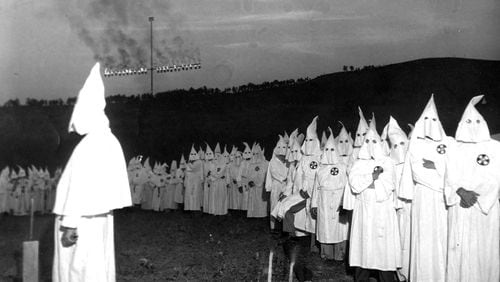This black and white historical photo captures a solemn, controversial gathering of Ku Klux Klan members arranged in a horizontal rectangle format. Approximately 60 to 100 members, clad in their infamous white robes and pointed hoods bearing an emblem on the right side, stand in a line. Their poses range from holding their hands clasped in front of them, down at their sides, or over their hearts. Dominating the scene, a large burning cross emits black smoke from its horizontal bar, casting an eerie glow against the grayish sky. In the background, the somber atmosphere is framed by sparsely wooded hills. Notably, a lone Klansman stands off to the left side of the image, gazing intently towards the burning cross.